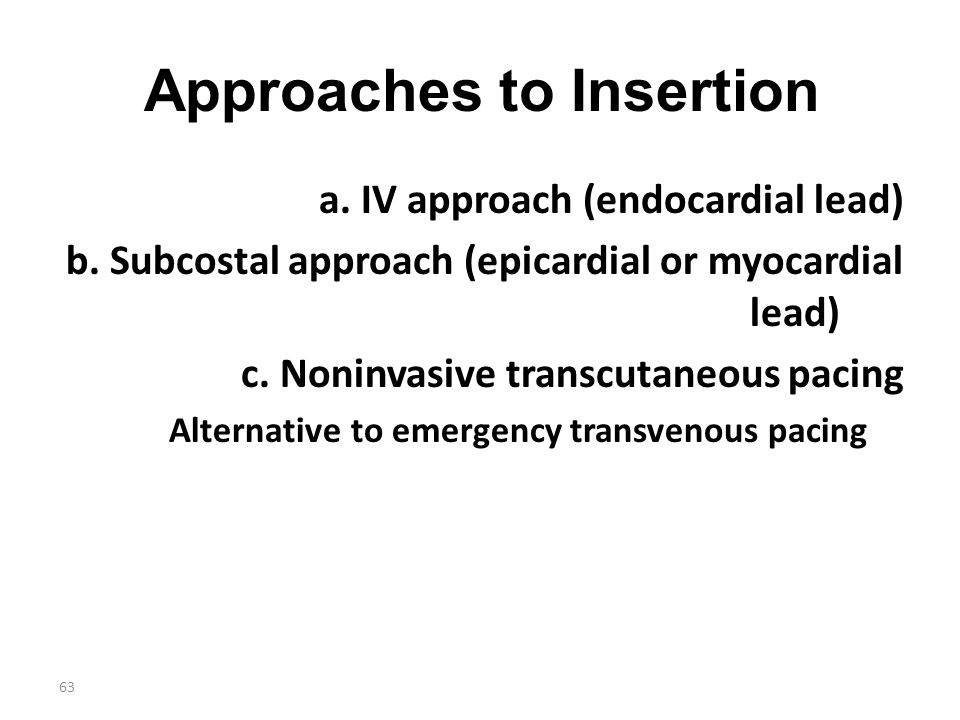The image is a black-and-white educational medical slide, designated as page 63 at the bottom left in gray font. The slide has a clean, simple design with right-aligned, unremarkable Arial font text on a white background. At the top, a bold headline reads "Approaches to Insertion." Following the headline, the slide lists several insertion methods, each starting with a lowercase letter in bold. 

- **A.** IV approach (endocardial lead)
- **B.** Subcoastal approach (epicardial or myocardial lead)
- **C.** Non-invasive transcutaneous pacing

Beneath these methods, in smaller text, it notes "alternative to emergency transvenous pacing."